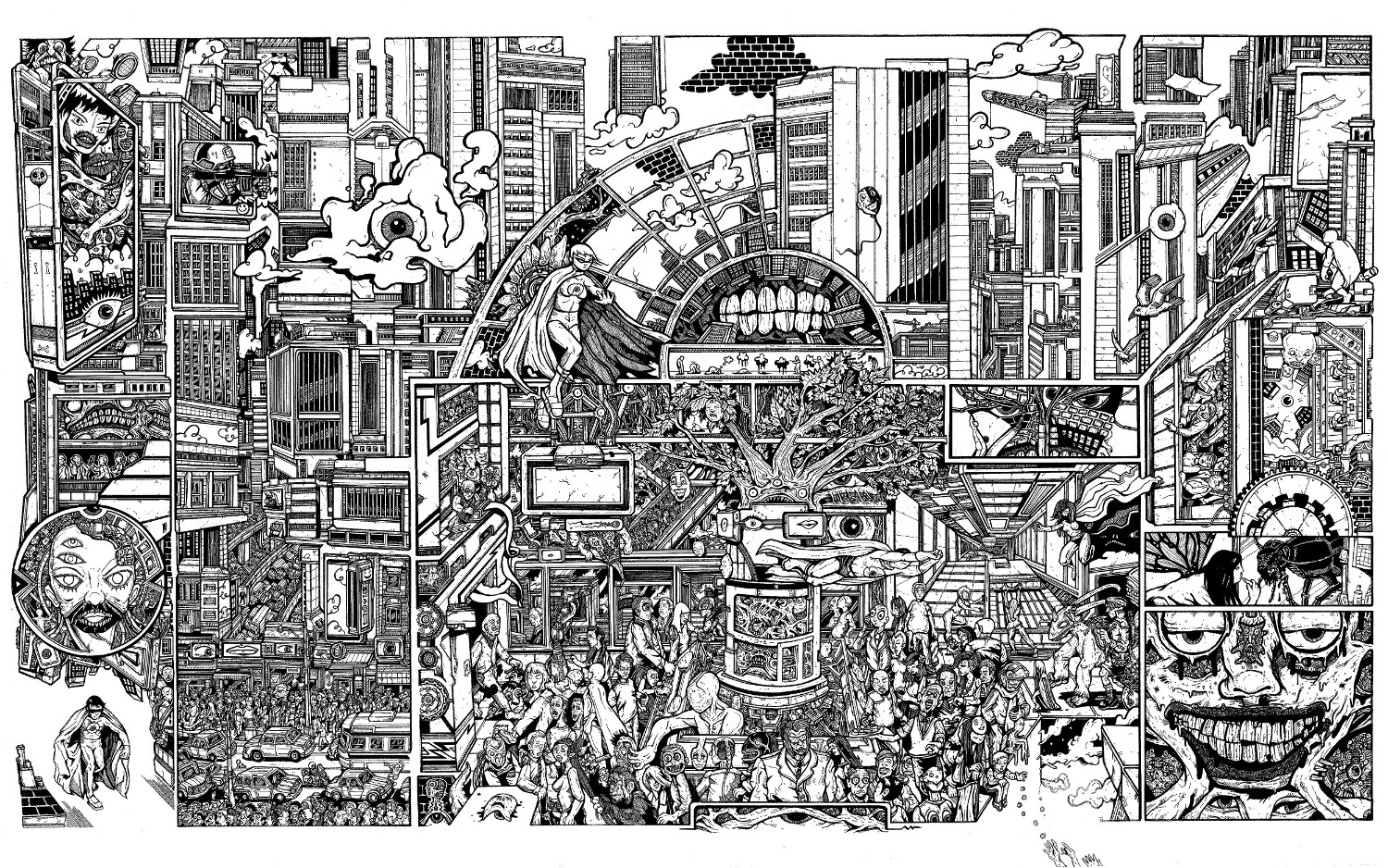This intricate black and white sketch on a rectangular white surface depicts an overwhelming array of detailed images, densely packed from edge to edge. The illustration spans much wider than it is tall and lacks any bare spaces, evoking a chaotic and eerie atmosphere reminiscent of a monochromatic, nightmarish "Where's Waldo."

Central to the unsettling composition is an array of grotesque faces, including a particularly disturbing one with a large mouth, sharp teeth, and big eyes, hands pressed against its cheeks. Nearby, a skeletal visage with black teeth adds to the macabre feel. The artwork features a diverse cast of characters—ghouls, mummies, naked figures, superheroes in capes, and what seem to be Super Marvel characters—seamlessly integrated into a busy cityscape.

Amidst the crumbling buildings with exposed brickwork and worn stucco, one can spot windows inhabited by eerie faces, ghouls, and bizarre figures. An arch in the center cradles black and white windows, from which lightning seems to emanate from a box below. Up above, there are clouds and birds adding to the frenetic sky, while an iPhone with an eye on its bottom lies in the upper left corner, surrounded by more faces and bodies. In the midst of all this, an elephant and a face appearing on a balloon adds an odd, surreal touch.

This highly detailed drawing, devoid of color yet rich in grayscale, is a testament to the artist's effort, filling every inch of the canvas with intricate and unsettling imagery. Each element, from the larger, prominent figures to the smallest, barely identifiable ones, contributes to the overall sense of a dark, crowded scene that is both fascinating and profoundly disturbing.